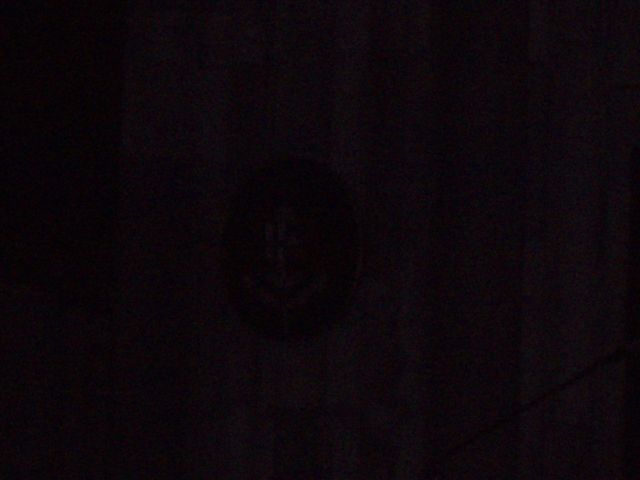The image is an expanse of unbroken darkness, offering no discernible shapes, colors, or objects. There is a subtle gradation of gray barely perceptible within the inky blackness, demanding a concerted effort to detect. Whether the image stems from a video game or an attempt to capture an elusive nocturnal moment remains unclear. The photo lacks any contextual clues, presenting a void devoid of text, setting, or stylistic elements. Neither human eyes nor Google's algorithms can decipher any hidden details. It is simply an image of profound and undisturbed night.